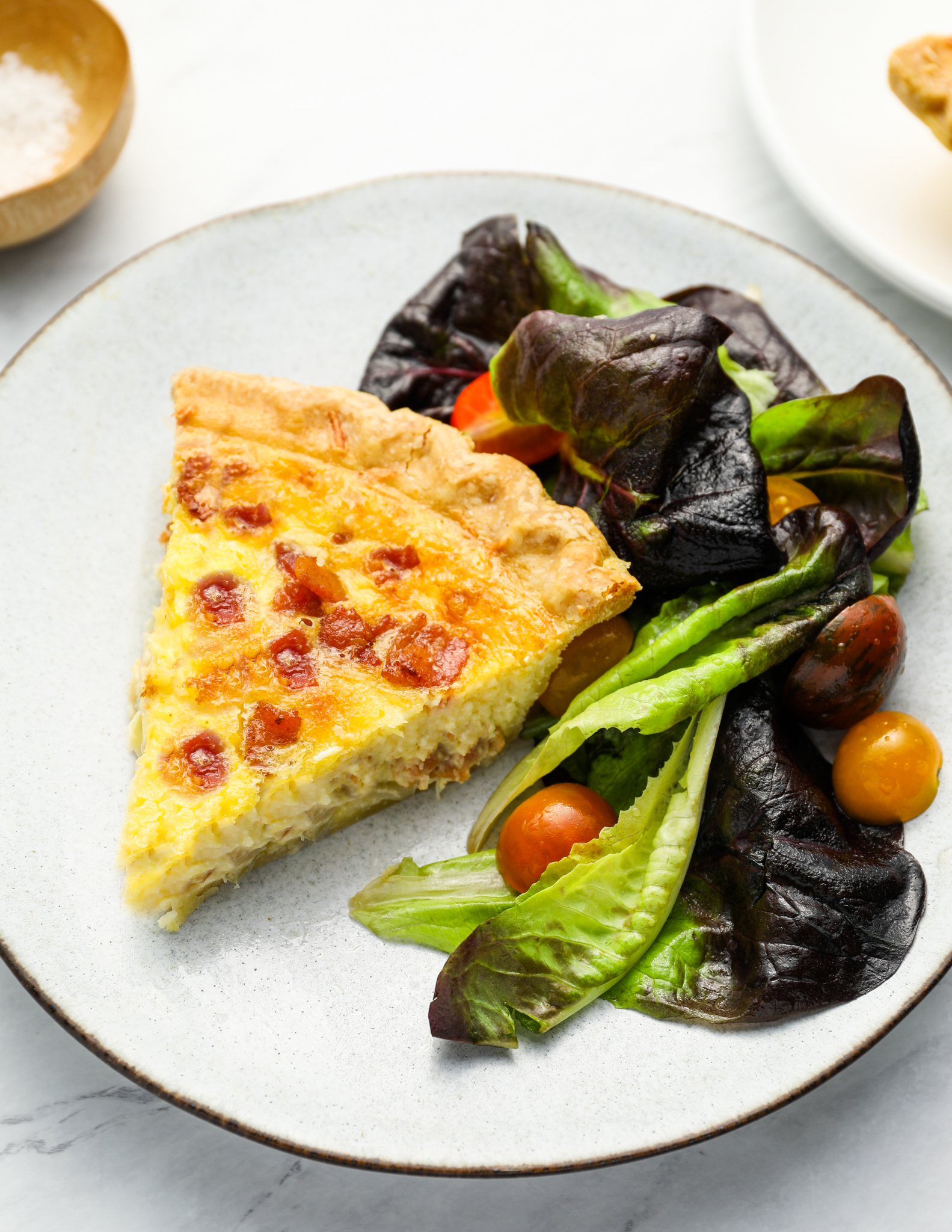The picture showcases a close-up of a meal set on a marble table, featuring a white plate with a distinct black outline. Centered on the plate is a slice of quiche, resembling a piece of pie with a perfect, unburnt crust, and topped with melted cheese and crispy bacon pieces. To the right of the quiche lies a vibrant salad composed of leafy greens, some of which are dark purple or black. Interspersed within the salad are small tomatoes in shades of orange, red, and purple, possibly dressed with a light oil. Positioned above the main plate is a small wooden bowl containing salt. In the top right corner, a second white plate with another piece of quiche peeks into view, maintaining the meal's thematic consistency. Remarkably, no silverware is present, and all the food remains untouched, emphasizing its fresh and appetizing presentation.